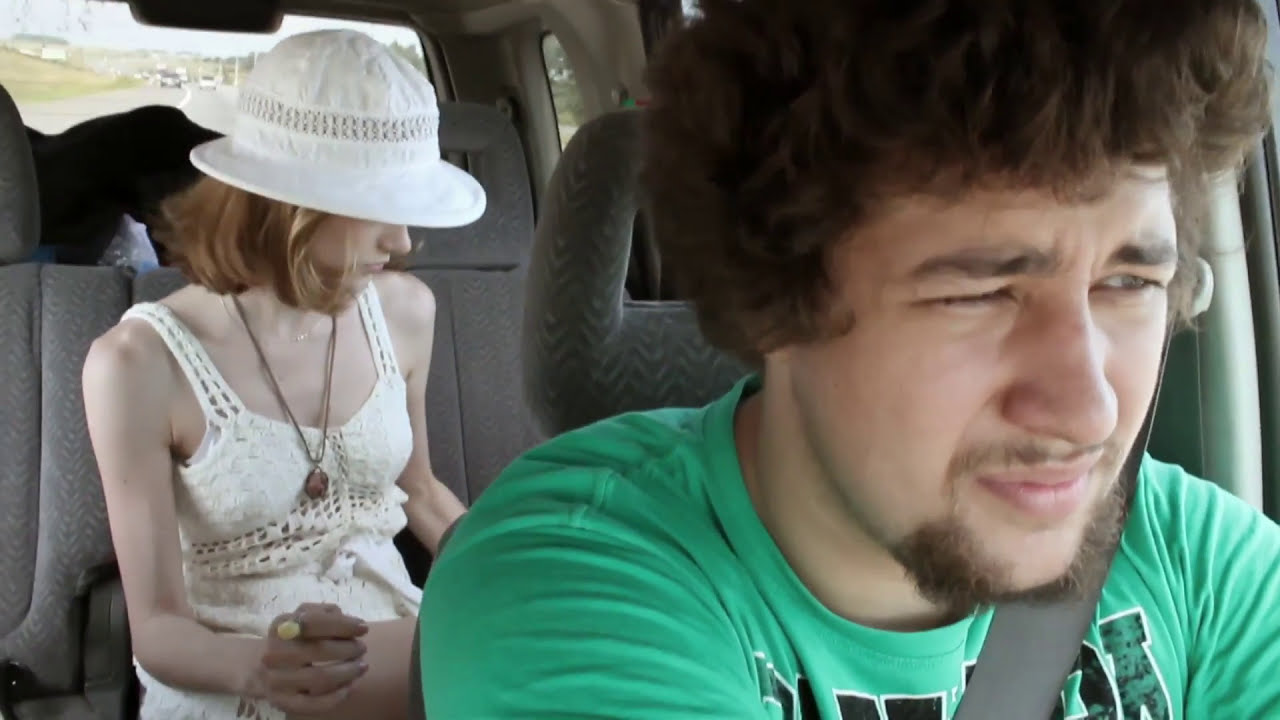In the foreground of the car's interior, a young man with curly brown hair, a beard, and a mustache grimaces as he looks forward, possibly concentrating on the road ahead. He's dressed in a green graphic t-shirt and is secured with a gray seat belt. Behind him in the passenger seat sits a woman donning a white bucket hat and a white dress. She has blonde hair and wears a brown necklace, her attention downwards to her left, possibly looking at a phone. In the cargo area positioned behind her seat, black luggage is visible. Through the rear window, a highway and several cars, set against a green landscape, stretch out in the distance. The vehicle appears to have a gray interior and is possibly a minivan. The scene captures a moment of focused travel.